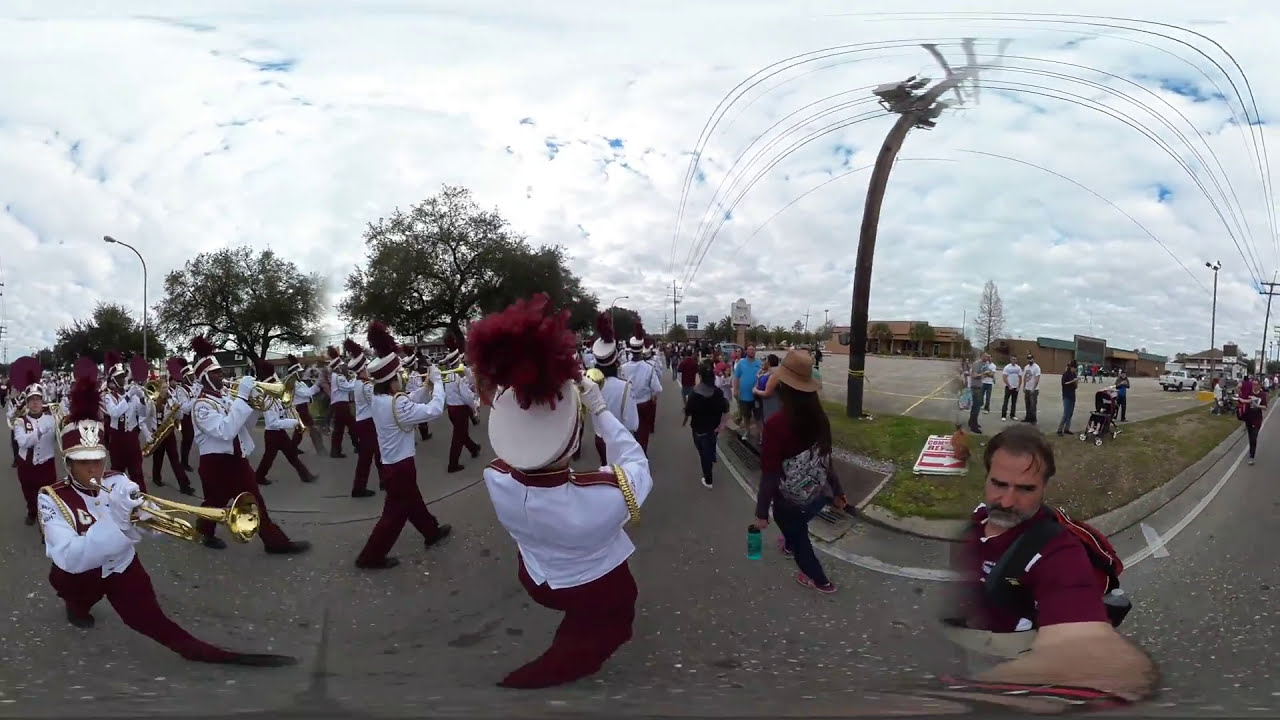This outdoor daytime photograph captures a visually striking and warped image of a marching band parading down a straight, paved road. The use of a wide lens and specialized effects creates a surreal scene where the band, dressed in matching white long-sleeve shirts with gloves, burgundy red pants, and decorative hats with furry feather tops, appears to stretch and curve unnaturally. On the far left, a band member's leg is elongated, while those in the center exhibit shorter, curved legs due to the distortion. On the far right, an older Caucasian gentleman with a gray mustache and beard, wearing a short-sleeved red polo shirt, stands with his left arm extended, although his hand is disproportionately large and merges blurrily with the background. The road bubbles and curves beneath the band and the photographer, accentuated by a bent telephone pole and a sky rendered wavy by the effects. The photograph also hints at an audience, with people standing in a parking lot on the right-hand side, observing the surreal transformation of the mundane march into a dreamlike spectacle.